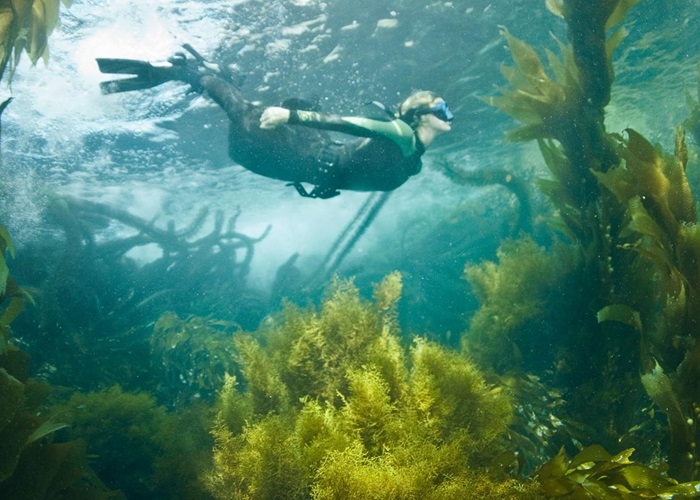This underwater photograph captures a serene diving scene featuring a woman immersed in an aquatic landscape teeming with marine vegetation. The diver, identifiable by her blonde hair, dons a gray-black wetsuit accented with green along the shoulders, a weighted belt to maintain depth, and black flippers. Her exposed hands are free to navigate through the clear yet slightly disturbed water. Despite the lack of a visible respirator or snorkel, she wears a protective mask over her face. The diverse underwater flora is prominently displayed, with lush towers of kelp and seaweed in shades of green and yellow stretching upwards, almost reaching the well-lit water's surface. Sunlight filters through, bathing the underwater scene in a light transparent blue hue, enhancing the visibility of the tall green plants with large leaves and the dense sea vegetation that surrounds her. Notably absent are any fish, leaving the focus on the rich, vibrant plant life and the peaceful diver exploring this underwater haven.